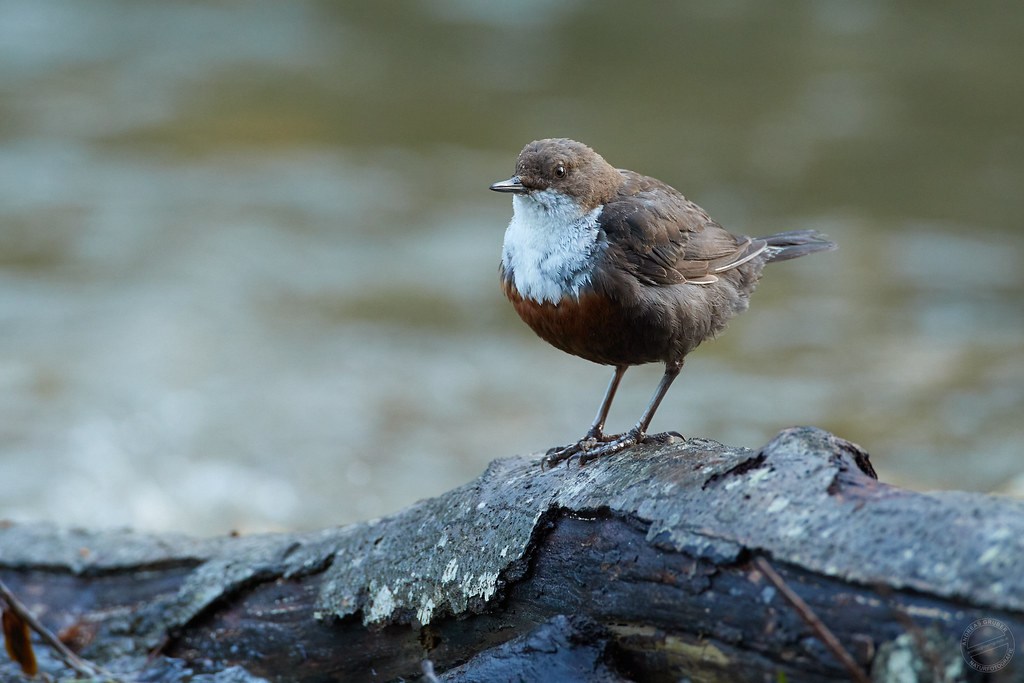In this close-up photograph taken outdoors during the daytime, a small, fluffy, stout bird is perched on a partially rotting log or fallen tree branch. The log, displaying a mix of brown, gray, and a hint of bluish tones in its bark, dominates the lower part of the image, creating a natural platform for the bird. The bird itself, with a round body and short black beak, is captured in crisp detail against a blurred, indistinct background that comprises dark brown, white, and faint blue tones.

This bird's brown head and back contrast with the white feathers extending from just below its beak down to its chest, blending into a reddish-brown belly. Its tail and wings feature predominantly dark brown feathers, with a hint of white on one feather. The bird is facing to the left, appearing very still and slightly to the side, allowing a clear view of its subtle feather details and the glint in its brown eye. Despite the overall darker tones of the photograph, the bird’s delicate features and the texture of the log stand out sharply, making it a vivid and striking image.